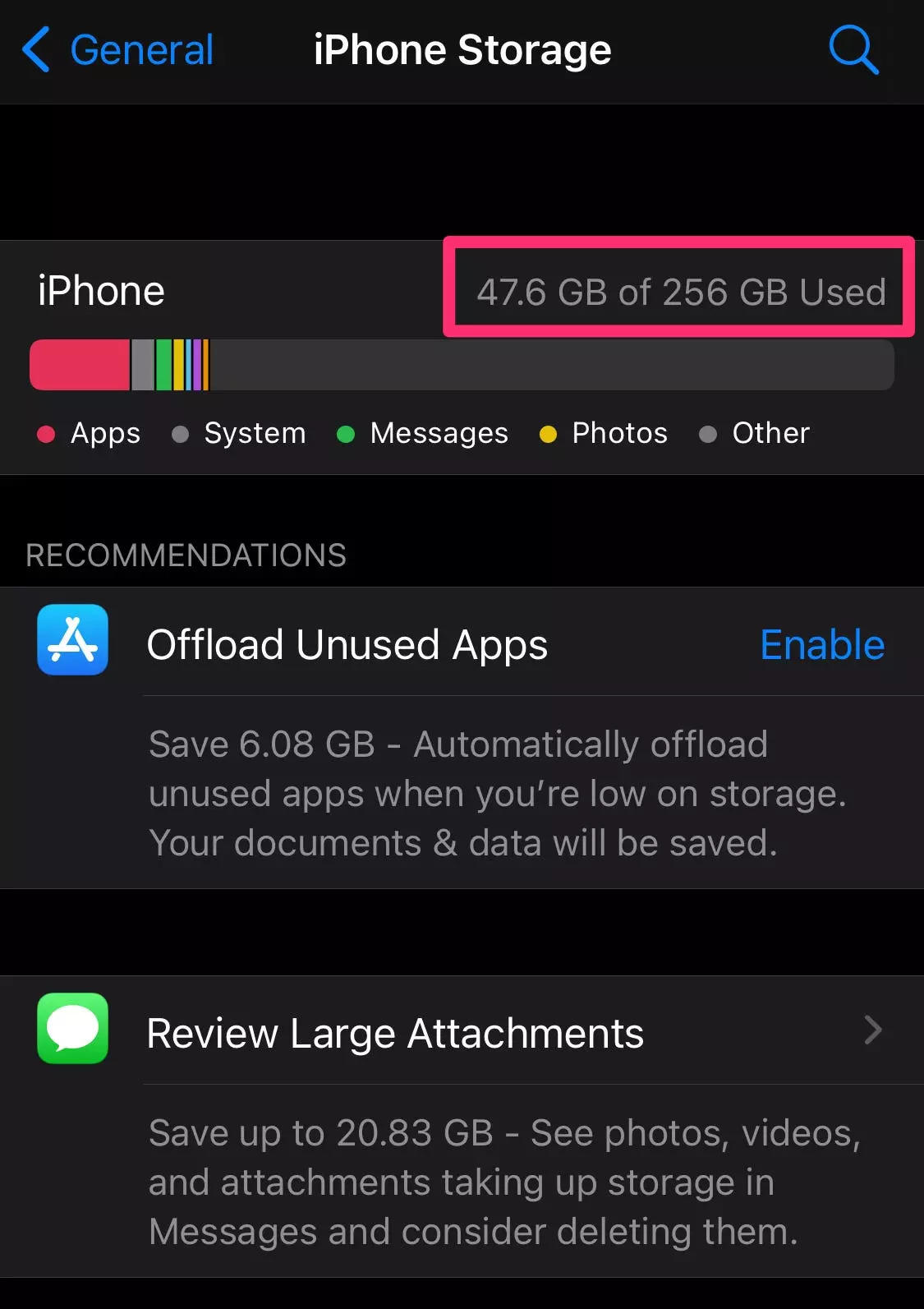A detailed screenshot of an iPhone storage screen is shown. At the top, a navigational back button is visible, accompanied by the blue text "General." Below this, the main header reads "iPhone Storage" next to a blue magnifying glass icon, all set against a light gray background, transitioning to a medium gray shade with a black bar beneath, before returning to gray once more. 

In the highlighted section, labeled "iPhone," it states that 47.6 GB of 256 GB are used, with "GB" signifying gigabytes. A large, color-coded bar visually represents the storage usage. The bar is segmented, showing red for "Apps" as the largest portion, followed by gray for "System," green for "Messages," yellow for "Photos," and another gray for "Other," with the sections progressively decreasing in size from left to right.

Beneath this bar is a black area titled "Recommendations." Here, a recommendation to "Offload Unused Apps" is displayed, featuring the App Store icon (a white "A" on a blue field) and an option to enable the feature, promising a saving of 6.08 GB. The description explains that unused apps will be automatically offloaded when storage is low, while documents and data associated with those apps will be preserved.

Further down, another recommendation suggests reviewing large attachments. This section, marked with a chat icon, indicates that up to 20.83 GB can be saved by reviewing and potentially deleting photos, videos, and attachments that are occupying storage within messaging apps.